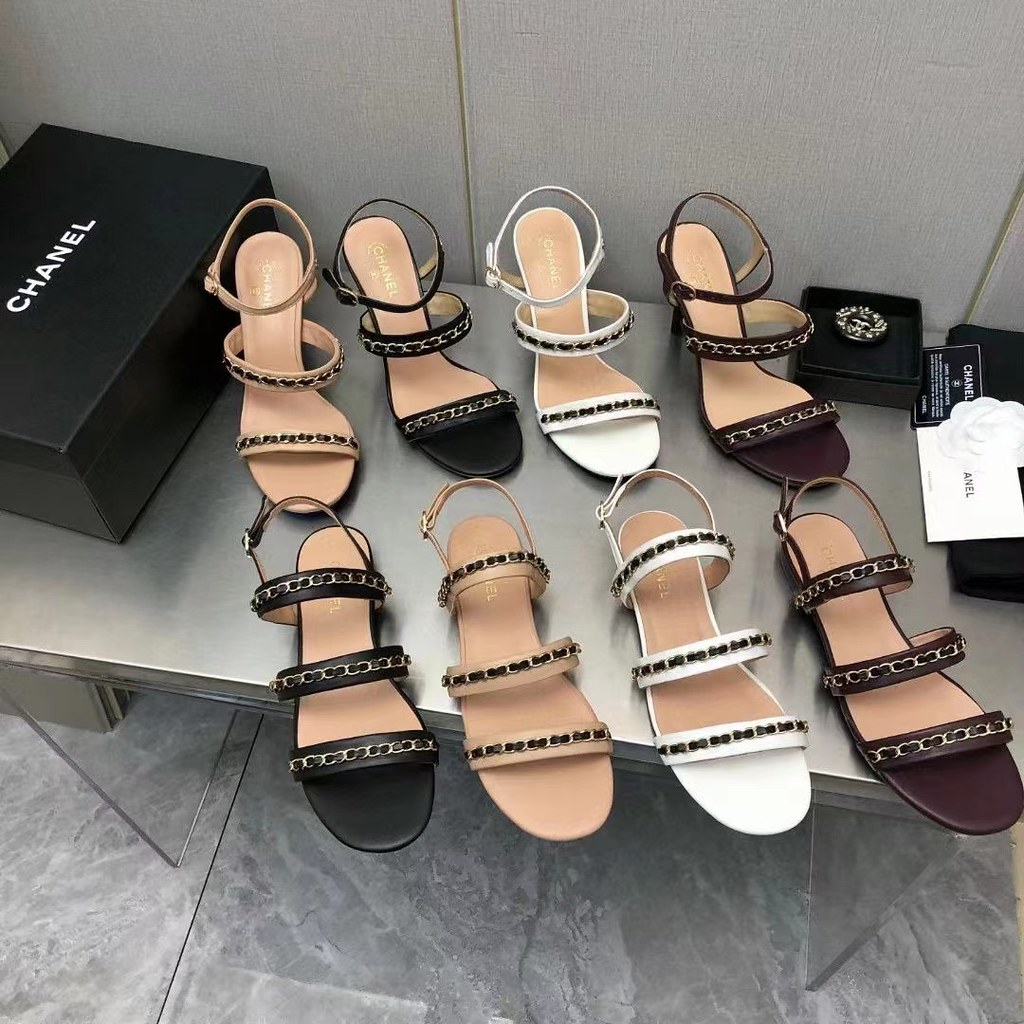The image showcases a selection of Chanel strappy sandals displayed on a shiny silver surface, which appears to be a seat for trying on shoes in a store. The floor beneath is sleek gray marble. Positioned on the upper left corner of the display is a black Chanel shoe box with white writing. Additionally, there's a small Chanel box, seemingly containing a metal brooch, accompanied by the brand's signature black and white card. The image features a total of eight individual right-foot sandals, organized by their different styles and colors. In the back row, there are four high-heeled sandals: tan with black detailing, tan with a black toe and some gold accents, white with black detailing, and a dark red pair with gold detailing. In the front row, matching flat sandals in the same colors are aligned directly in front of the corresponding high-heeled versions, except for the tan and black ones, which are switched. The arrangement elegantly displays the variety in colors and styles offered by Chanel.